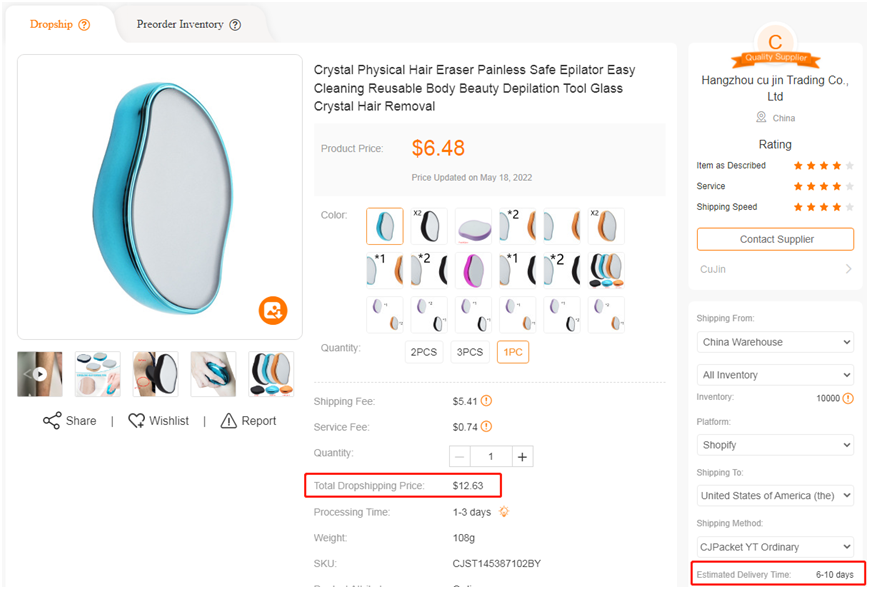**Caption:**

A detailed screen capture from Alibaba displaying a product listing for the "Crystal Physical Hair Eraser." The website features a light gray background with white text areas and black text, complemented by bright orange accents. The primary image showcases the product in a striking metallic blue, accompanied by additional thumbnails displaying its use and various color options (blue, black, purple, pink).

The product, described as a "Painless Safe Epilator Easy Cleaning Reusable Body Beauty Depilation Tool," is priced at $6.48 (updated on May 18, 2022). Available in quantities of one, two, or three, the product incurs a shipping fee of $5.41 and a service fee of $0.74, bringing the total drop shipping price to $12.63. Red boxes highlight specific information, including seller details on the right side and the estimated delivery time of six to ten days.